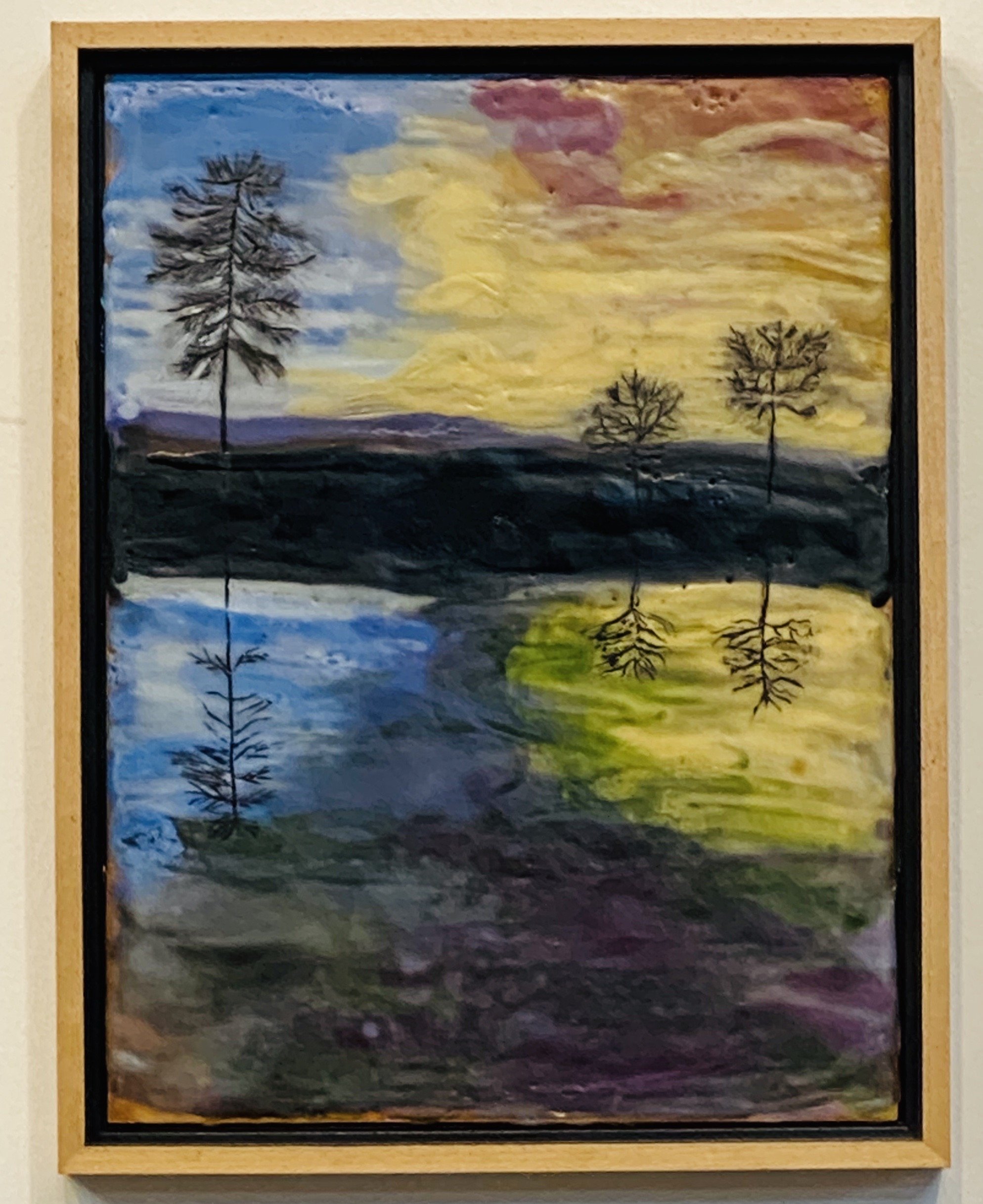This framed painting appears to be an acrylic or watercolor piece characterized by its rudimentary yet intriguing texture, possibly featuring areas of thick paint or damage. The artwork is set in a light wooden outer frame with a darker inner frame and depicts a serene landscape split horizontally by a dark strip of land. On the left side stands a sparse, scraggly pine tree, while the right side showcases two slender, branchless trees. The background sky transitions from blue and white on the left to a gradient of yellow, orange, and red on the right, mirrored in the water below. The reflections in the water are imperfect, with the left tree and the right-hand trees missing some branches in their mirrored images. This captivating depiction blurs the line between natural scenery and abstract art, encapsulating both earthy and vibrant hues.